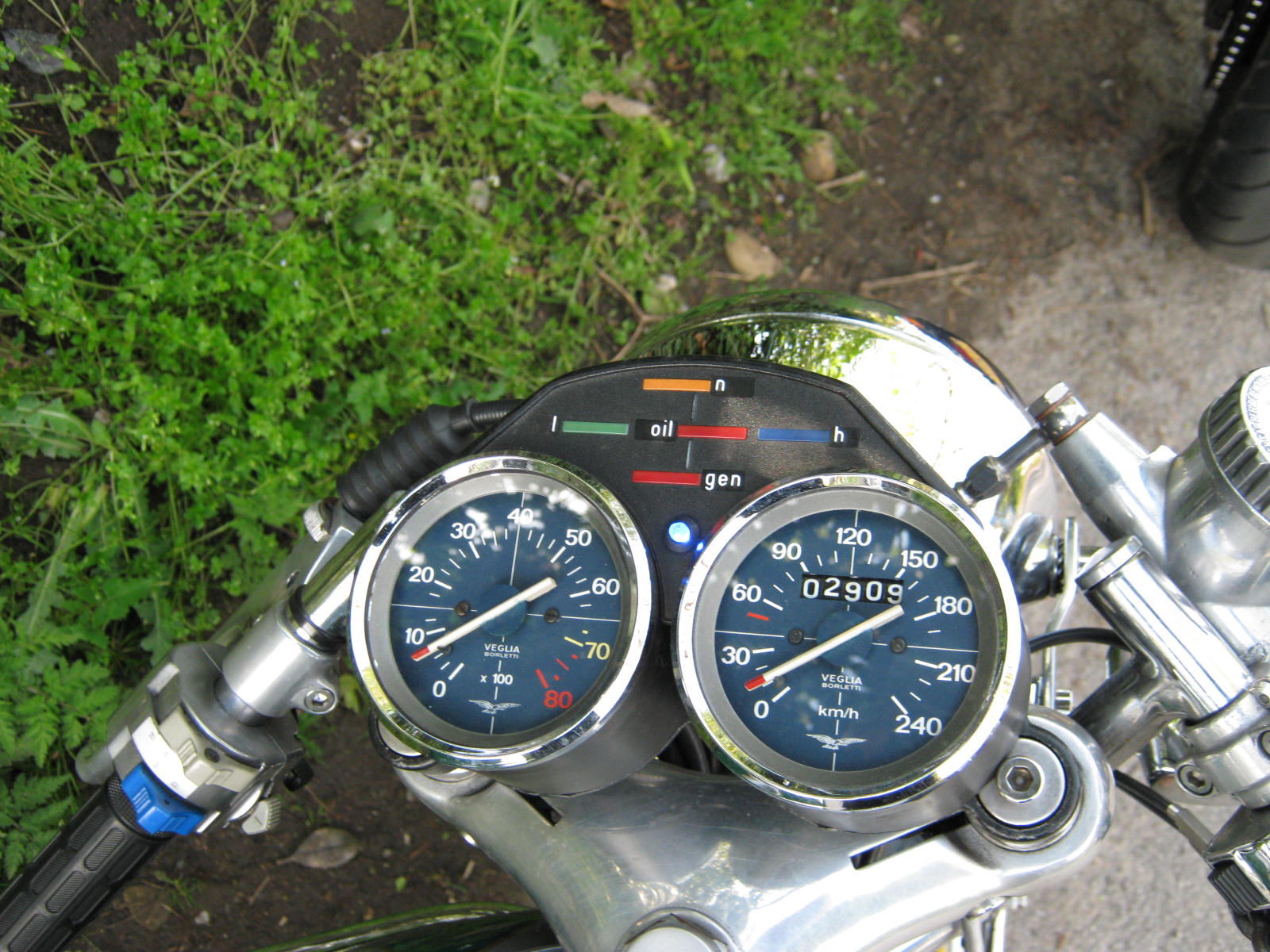Aerial view photograph of a silver and blue motorcycle, captured in landscape orientation. The motorcycle occupies the bottom portion of the image, showcasing its sleek design with a white base. Prominently visible are two gauges side by side, featuring dark blue backgrounds with white fonts. The motorcycle is parked on a gray concrete surface. In the top left corner of the image, light green shrubs add a touch of nature. The top right corner reveals a mysterious black object adorned with a vertical line of white circles.